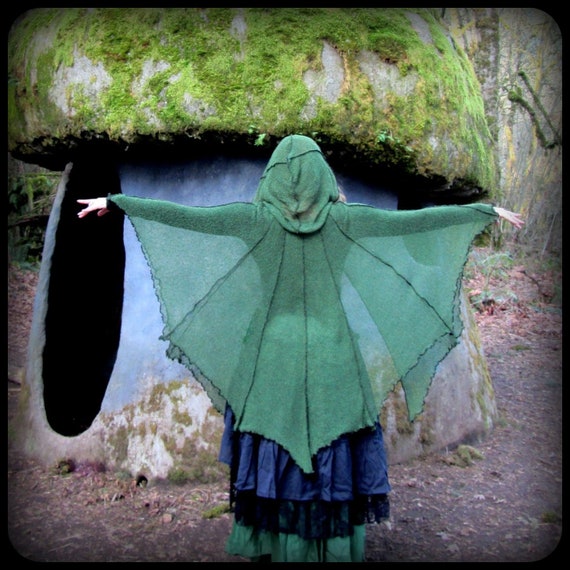The photo features a woman with light skin standing in a forest, her back to the camera, and her arms extended wide horizontally as though embracing the scene. She is dressed in traditional attire with a green, translucent veil and headscarf, resembling wings as it drapes down to her blue skirt, which has several tiers including a purple one with black lace and a matching green layer underneath. The image exhibits a black outline fading towards the edges, adding an ethereal quality. In front of her stands a whimsical, stone hut with a curved, moss-covered roof, bearing a reminiscent appearance of a mushroom or yurt. The structure has an oval opening on the left and sits amidst a clearing in the woods, suggesting an old and mystical atmosphere. The overall impression is one of an enchanting, fairy-tale scene designed for a personal photo book or social media, blending traditional beauty with natural, rustic elements.